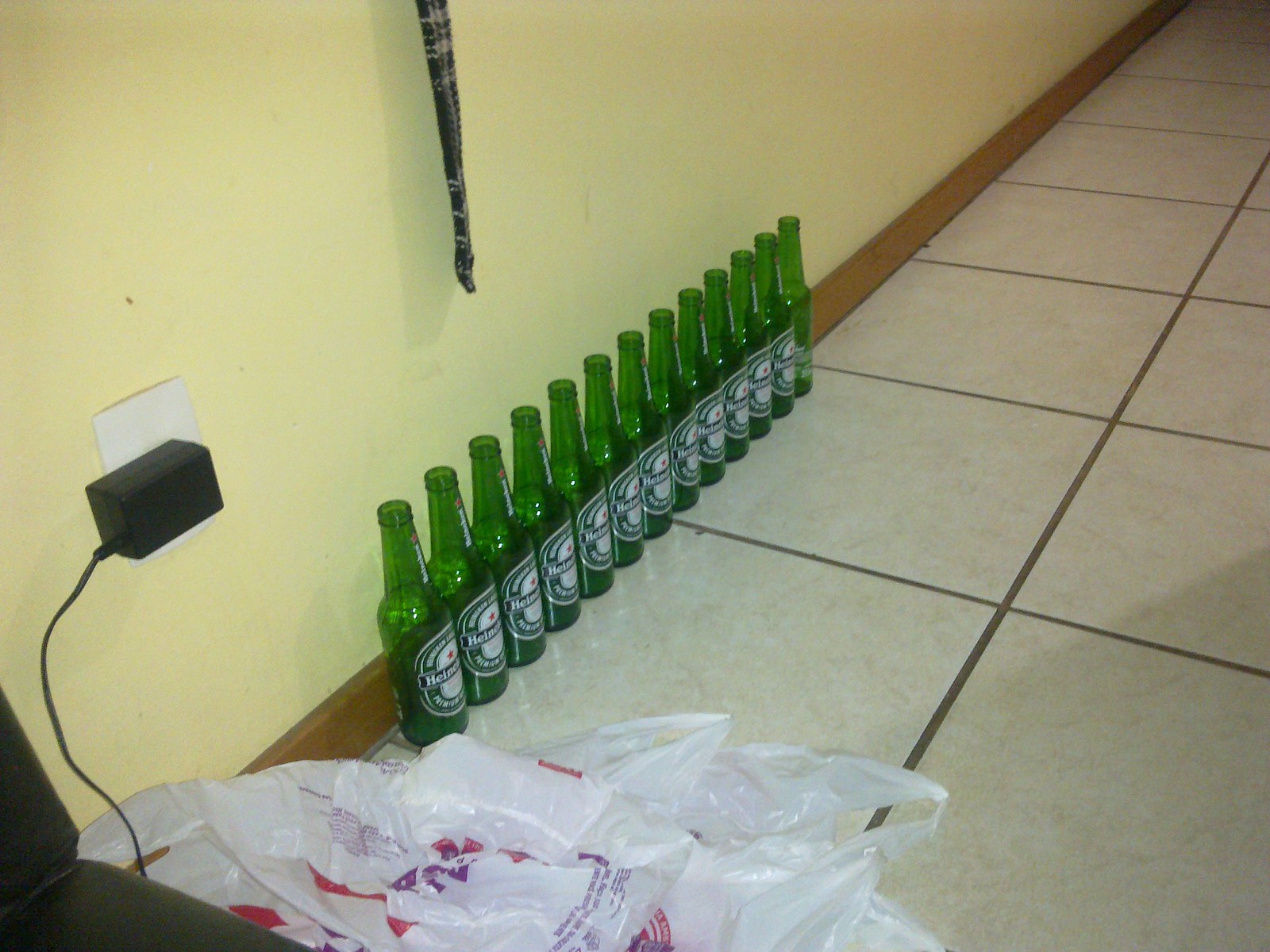This dimly-lit, grainy indoor photograph captures around 15 green Heineken beer bottles, each adorned with the classic Heineken logo, neatly lined up against a banana-yellow painted wall. The bottles rest on large white kitchen tiles. An electrical outlet on the wall has a black device, possibly a charger, plugged into it. Nearby on the floor, a pile of plastic grocery bags is visible. A skirting board, made of wooden trim, runs parallel to the row of bottles. There's also a black leather seat partially visible in the frame, and a piece of fabric, resembling a tie, hangs down about a foot above the bottles, though its origin is unclear. The scene suggests a casual, perhaps slightly cluttered, home or rental setting.